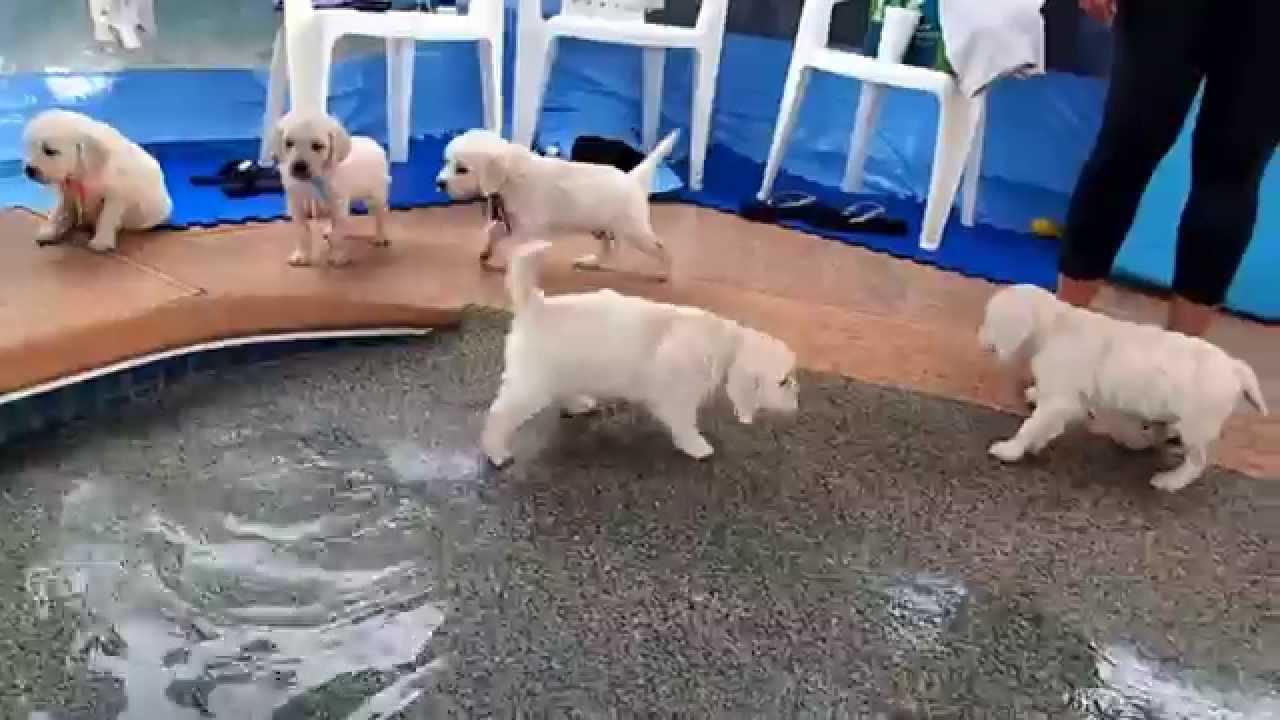The photograph captures a grainy, pixelated scene that appears to be taken at a dog park or a specific area designed for dogs. In the foreground, there is a small, uneven water pad or shallow doggie pool, featured prominently with clear, waterish hues. The pad is surrounded by five light-colored puppies that resemble golden retrievers or yellow Labrador retrievers. Three of these puppies are positioned on a beige-brown pathway that borders the water pad, while the other two puppies occupy the water, one wading through and the other standing at the edge.

To the right side of the image, a human figure, partially visible with legs clad in black pants, stands near three white plastic chairs. The overall color palette includes grays, blues, lighter blues, whites, blacks, beige, and touches of yellow. This setting, likely a dog park or a designated spot for dogs to play, vividly captures the playful yet serene interaction between the puppies and their environment.